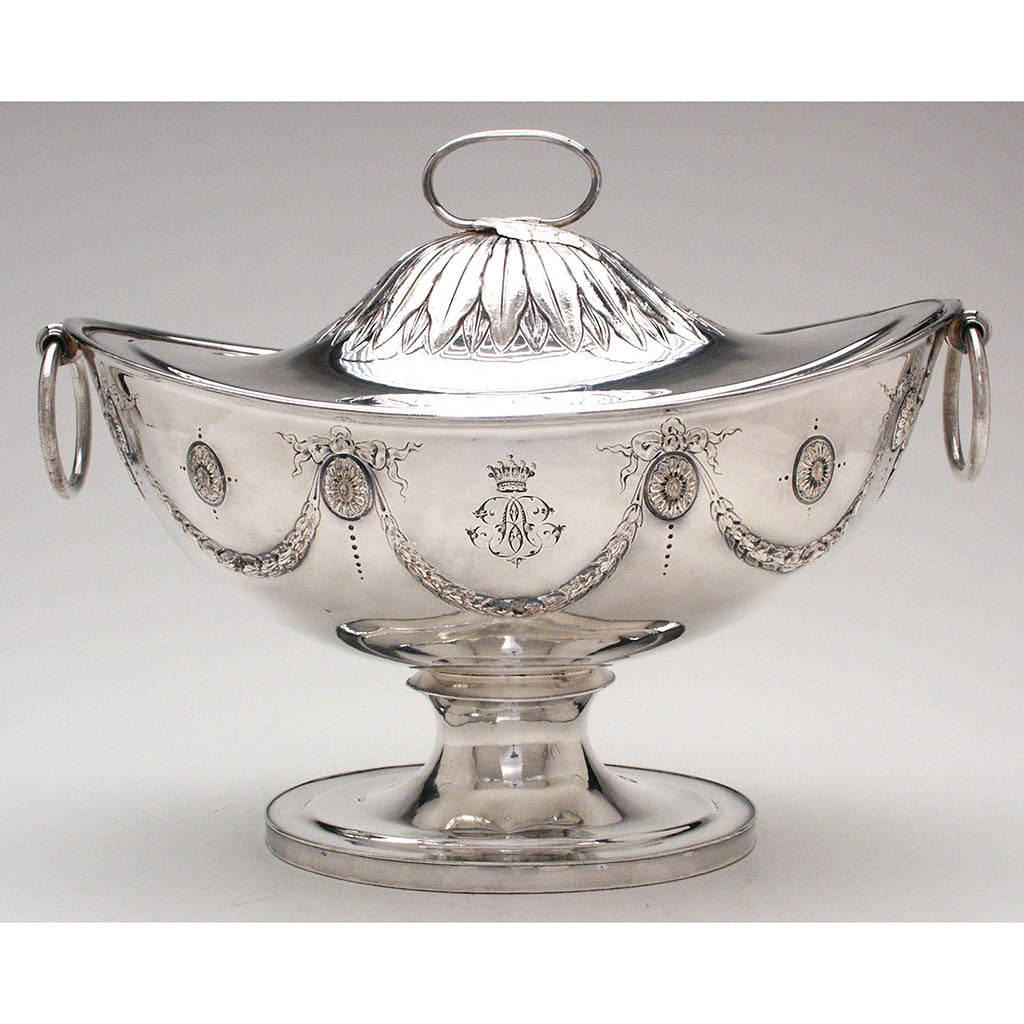This image showcases a highly ornate silver object with a gray background that transitions from a darker shade at the top to a lighter one at the bottom. The object resembles a genie lamp or a decorative household item, possibly an antique food holder used in banquets. The lid features an ovular handle and takes on the shape of a top hat. Intricately designed, the body of the object has an elaborate pattern that includes four circular motifs, each encircled by what appears to be woven or braided designs. At the center of these decorations, there is a prominent crown engraving, suggesting nobility or opulence. The object has two rings on either side, likely for carrying, and sits on a narrow, circular base that would rest evenly on any surface.